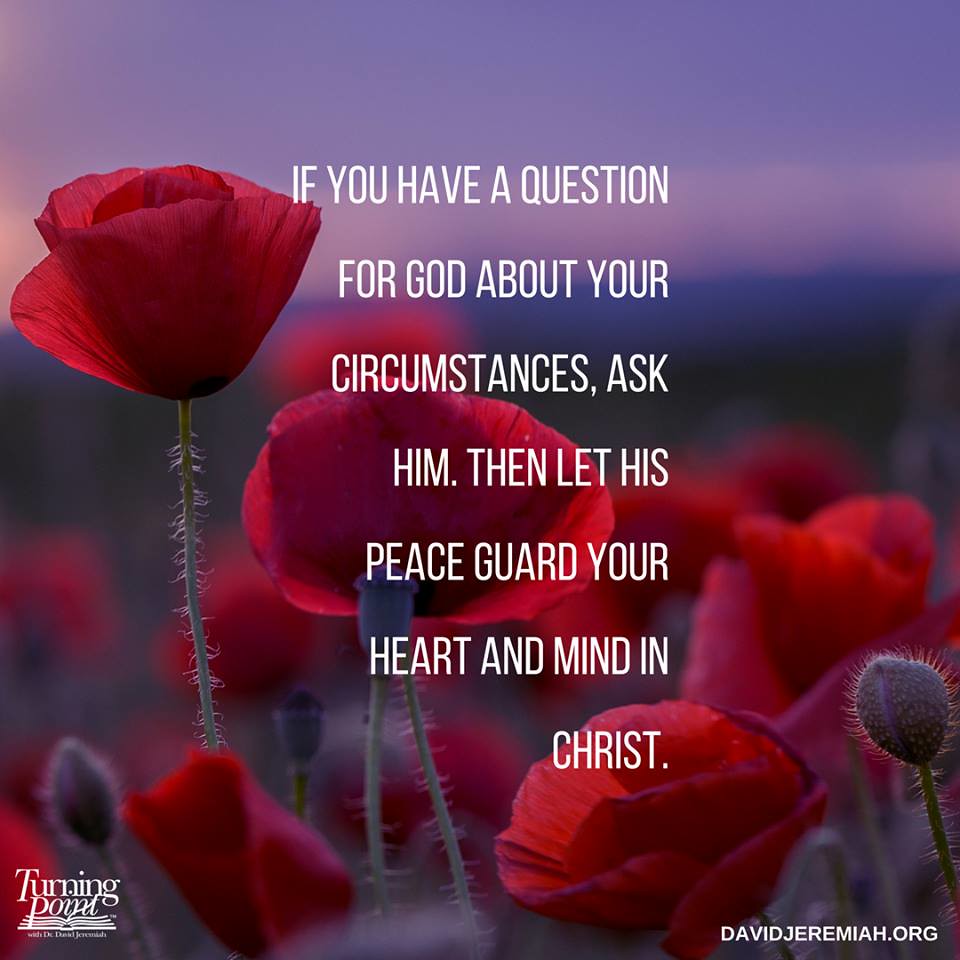The image is an inspirational poster featuring a vibrant, close-up photograph of bright pink, rose-like flowers with long, slightly fuzzy green stems. Towards the bottom right-hand side of the image, there is a budding flower on a stem that has yet to bloom. The composition of the flowers appears to increase in size from right to left, ascending higher into the air. The background is predominantly blurry with amorphous shapes of more red flowers, suggesting a field. In the distance, there is a mix of green land and a sky transitioning from light blues and purples, possibly indicating dawn or dusk. Overlaying this serene scene, in white uppercase text at the center of the image, is the quote: "If you have a question for God about your circumstances, ask Him, then let His peace guard your heart and mind in Christ." The bottom left-hand corner displays the "Turning Point" logo, along with an open book symbol underneath it, while the bottom right-hand corner features the URL "davidjeremiah.org."